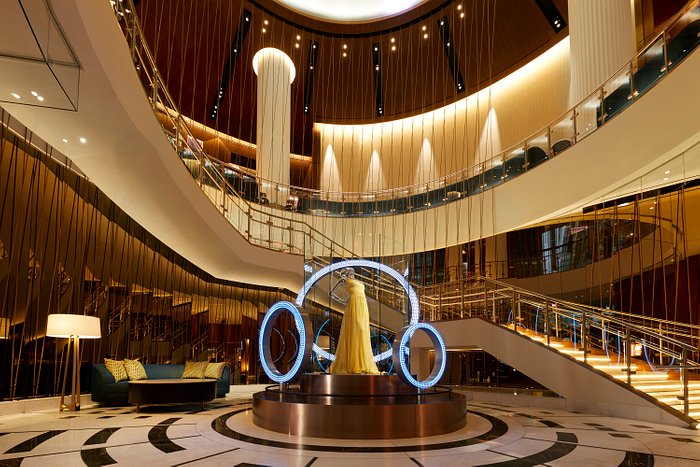This image captures a luxurious atrium inside a grand cruise ship, characterized by an opulent and ornate design. The expansive space is dominated by large white columns and rich brown wooden accents that adorn the walls and ceiling. Recessed lighting in some of the walls casts elegant triangular beams of white light down the cream-colored surfaces. The floor and grand staircase are crafted from a striking combination of white and black marble, with the staircase featuring golden railings that add a touch of regal elegance.

The central focal point of this atrium is a display art piece prominently positioned on a goldish-bronze pedestal with two tiers. The upper tier supports a glass-type figure adorned in an off-white, floor-length dress, while several chrome rings with blue illuminated edges encircle the figure. These rings are as tall as the dress, creating a visually captivating centerpiece.

At the lower level, a cozy seating area is visible, featuring a couch and a coffee table accompanied by a lamp. The illuminated steps of the staircase further enhance the grandeur, and the abundant cream and brown color palette, along with a hint of mirrored gold paneling on the lower walls, contribute to the overall luxurious atmosphere of the space. The atrium has multiple levels, with the second tier displaying chairs and additional lighting, including a prominent central light fixture that further accentuates the room's splendor.